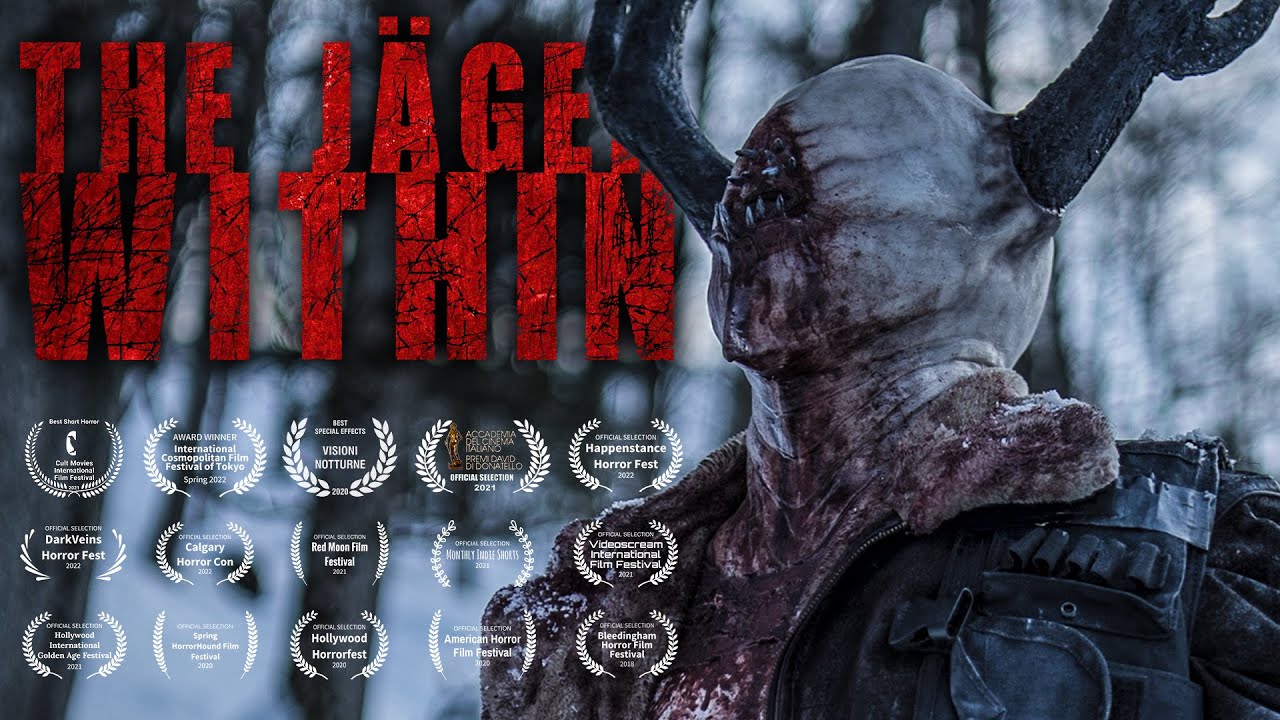The image is an advertisement for a horror movie titled "The Jäger Within," with the name written in striking red font, complete with black scratches and an umlaut over the "A," set against a dark grayish muted background that appears to include black tree silhouettes. Dominating the right side of the image is a nightmarish creature, depicted in a side view. This entity resembles a humanoid figure with antlers or horns protruding from either side of its head, wearing a leather tactical jacket layered with pockets and a wool collar stained with blood. Its face is horrifyingly devoid of eyes, nose, and ears, featuring only a grotesque, triangular mouth with outward-pointing teeth. The creature's veiny, pale complexion adds to its menacing appearance. 

In the lower left corner, we see numerous logos and accolades, 15 in total, celebrating the film's recognitions at various film and horror festivals. Some of these accolades come from the Hollywood Horror Fest, Dark Vein Horror Fest, and Happenstance Horror Fest, with others too small to read clearly. The overall atmosphere of the image is ominous and foreboding, effectively conveying the film's horror theme.